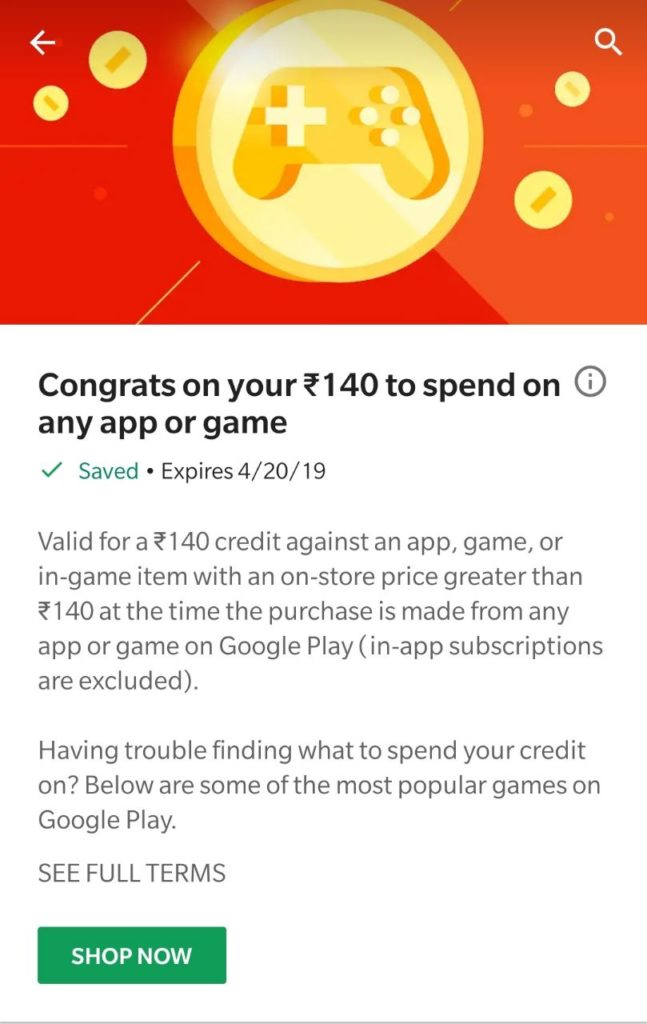The image displays a reward notification, featuring a vibrant and eye-catching design. At the top, there is a central image of a gold-colored Xbox controller, resembling a three-dimensional golden coin, against a rich red background adorned with yellow circles. Below the image, bold text exclaims, "Congrats on your $140 to spend on any app or game!" A zig-zag symbol accompanies the $140 amount for a stylish touch.

Further details specify the nature and terms of the reward. The text reads: "Saved. Expires 4-20-19. Valid for $140 credit against an app, game, or in-game item with an on-store price greater than $140 at the time of purchase made from any app or game on Google Play, in-app subscriptions excluded." This ensures clarity on how the credit can be used. 

For those needing suggestions, the notification helpfully adds, "Having trouble finding what to spend your credit on? Below are some of the most popular games on Google Play." To assist users further, the text encourages them to "SEE FULL TERMS" and features a prominent green button labeled "Shop Now" for immediate action.